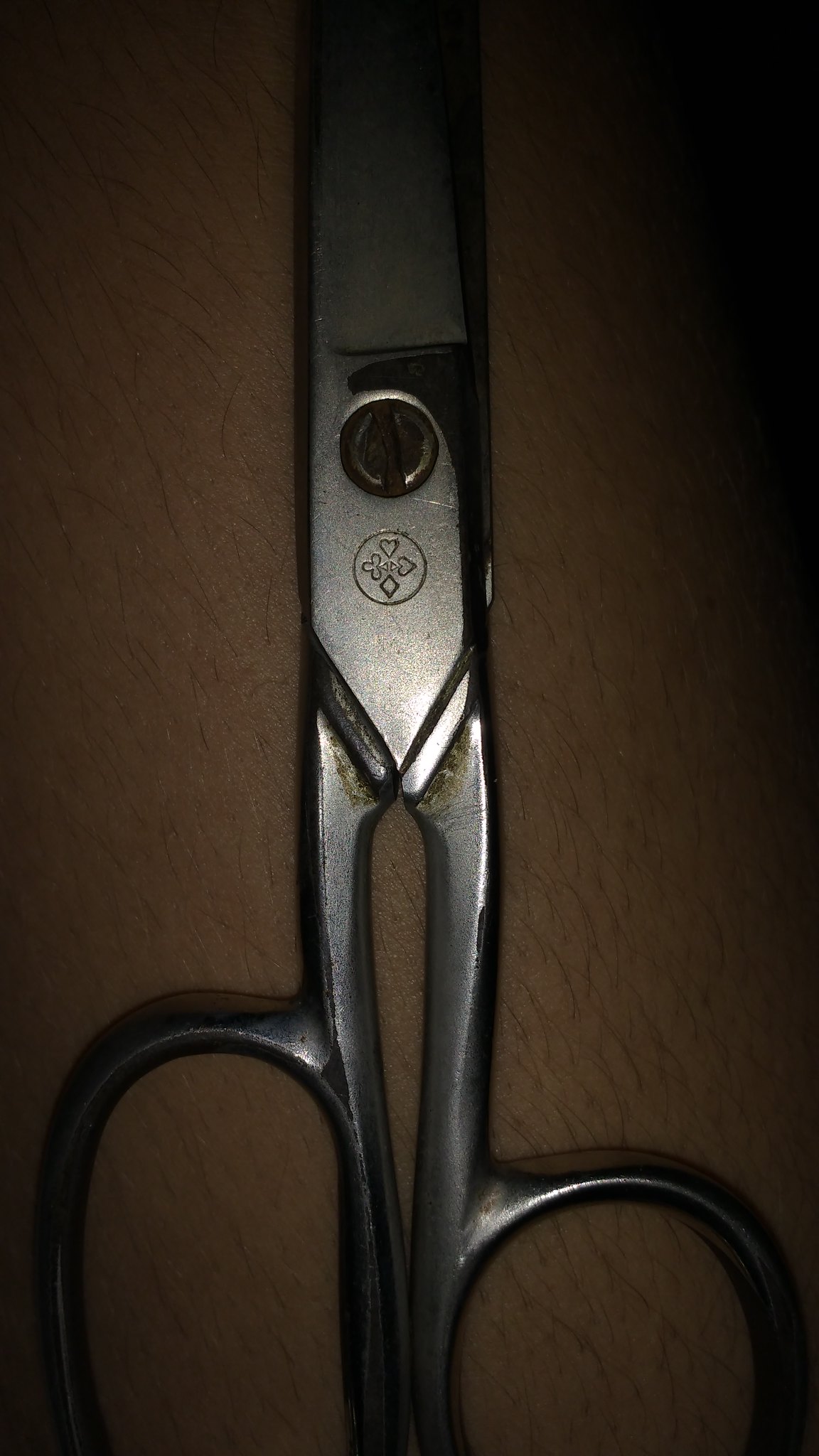This close-up photograph features a detailed view of an older, heavy-duty pair of steel scissors set against the pale skin of a person's leg, with noticeable dark leg hair visible. The scissors, which are vertically oriented with the tips and lower handle cropped out, exhibit signs of wear, including smudges and a pitted, steel gray handle. The finger holes are round, suggesting they might be old surgical scissors. The center of the image highlights a screw that holds the blades together, coupled with an oval engraving displaying a pinwheel-like decoration consisting of suits of cards—heart, diamond, clover, and spade. The backdrop is a brown surface, lighter in the center and darker at the edges, enhancing the scissors' gritty texture.